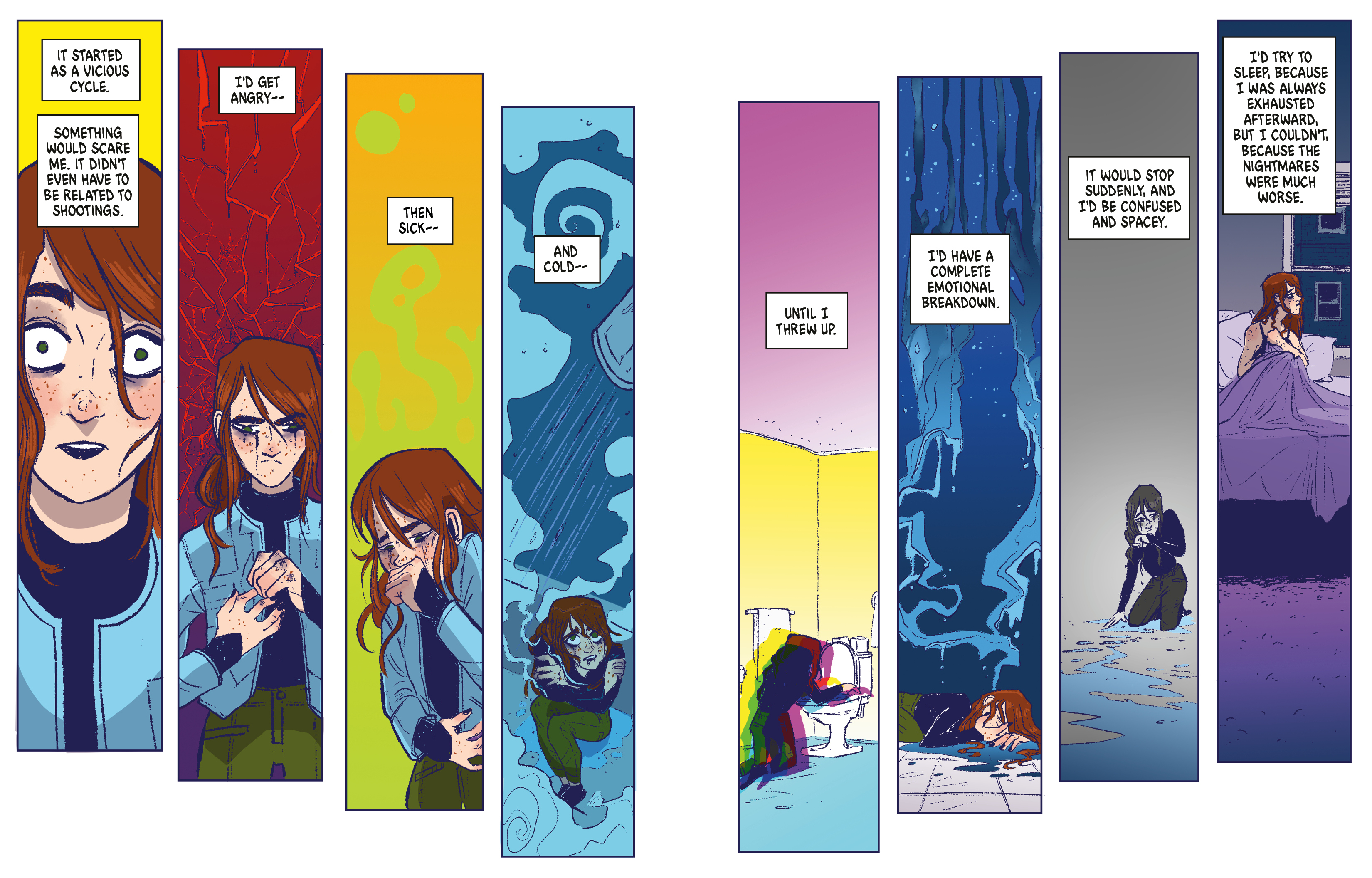This comic strip features eight vertical panels, each depicting a different stage in the life of a woman with long, scraggly reddish-brown hair, big eyes, and freckles. She is dressed in green pants, a blue turtleneck sweater, and a lighter blue jacket. Each panel is accompanied by a white text box with black lettering, narrating her emotional journey. The sequence begins with the woman looking forward, her expression reflecting a beginning phase, with text reading: "It started as a vicious cycle. Something would scare me. It didn't even have to be related to shootings." In the second panel, she stands with her hands out in front of her, illustrating anger and distress as the text explains: "I get angry and then sick and cold until I throw up." Subsequent panels show her progressively breaking down: in one, she appears to be coughing with her hand up to her face; in another, she is sitting surrounded by a bluish hue. The following panels depict her leaning over a toilet, lying on a tile floor with a blue background, kneeling as if there's water on the floor, and finally, sitting up in bed under a purple blanket, looking exhausted and facing right, with the text detailing her emotional and physical struggles culminating in confusion, exhaustion, and restless sleep plagued by worse nightmares. The entire sequence vividly portrays her distress and cyclical emotional turmoil.